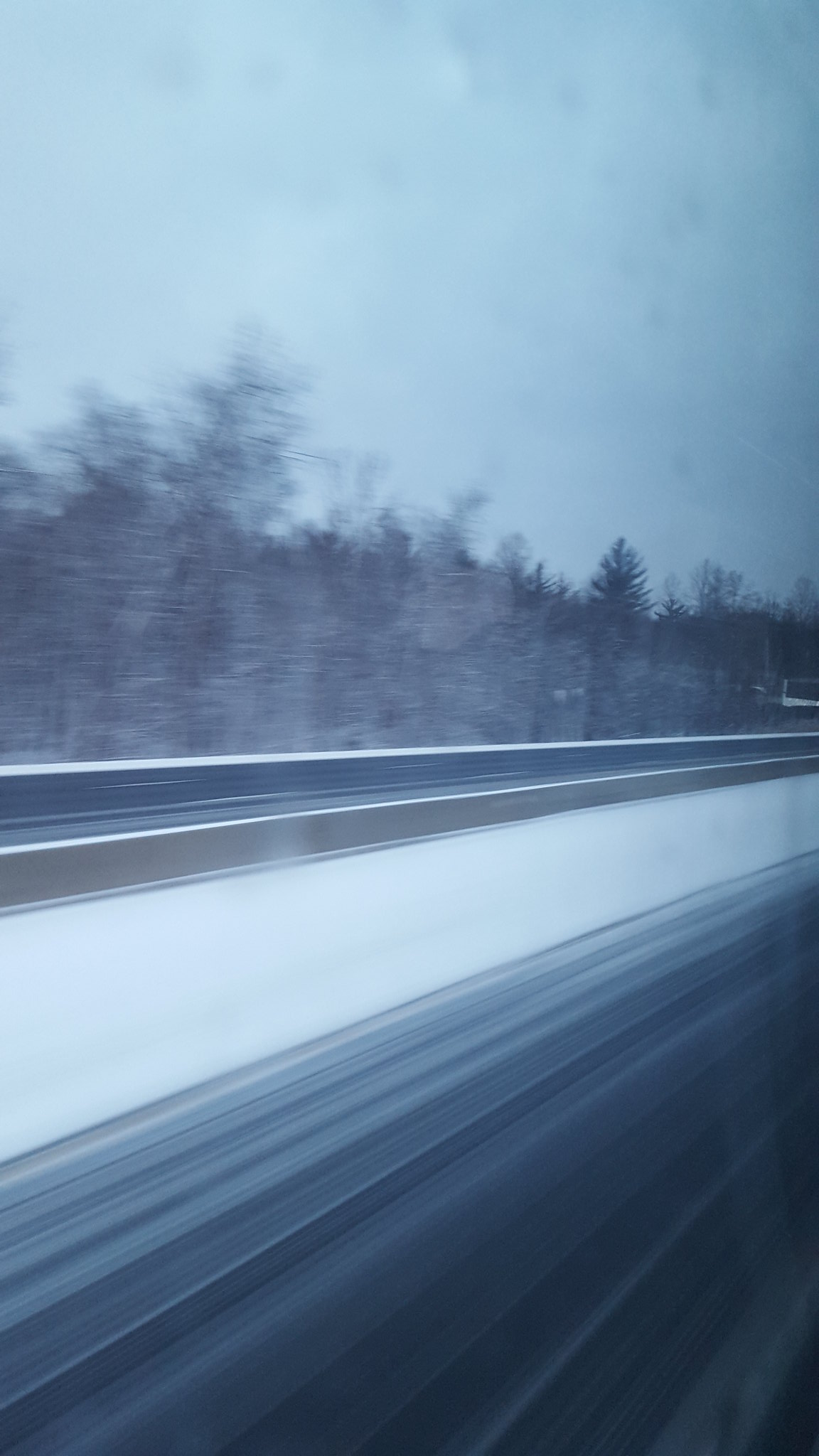A view outside a vehicle window captures a wintry landscape in motion. The large window frame, potentially emphasized by the photo's angle, provides a broad perspective of the scene outside. The road, slightly blurred due to the moving car, runs parallel to a snow-covered median, separating it from the opposite lane. Beyond this, a dense forest of tall trees stands majestically, their dark silhouettes contrasting with the snowy ground. The sky above is a muted grayish-blue, indicative of an overcast day, which imparts a cool, serene tone to the entire photograph.